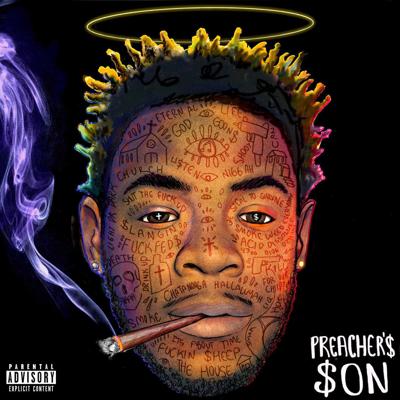The image is a CD cover set against a black background. It features a black man with intricate facial tattoos rendered in red ink, including words like "eternal," "god," and "goons," along with a small red cross on the tip of his nose and an eye on his forehead. His spiky black hair has tips highlighted in teal, yellow, and pink, and above his head, there is a thin yellow halo. He is smoking a joint, with purple and white smoke drifting upward. In the bottom left corner, white text reads "Parental Advisory Explicit Content," and in the bottom right corner, "Preacher's Son" is written in white font, with the S's replaced by dollar signs.